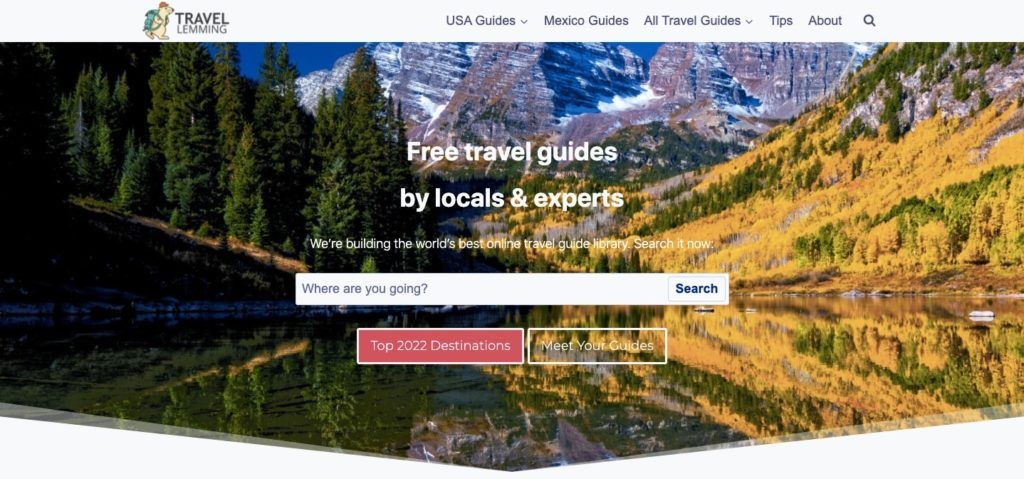This image, sourced from the Travel Lemming website, features a whimsical lemming dressed in a red hat and carrying a backpack. The lemming appears to be in motion, with one foot raised as if stepping forward. Surrounding the lemming, several drop-down menus are visible, labeled "US Guides," "Mexico Guides," and "All Travel Guides." Additional navigation options include sections for "Tips," "About," and a search function represented by a magnifying glass icon.

Dominating the screen is a large scenic photograph of a landscape with a water body, likely a large lake or pond, flanked by diverse terrain. In the distance, snow-capped mountains tower over the scene, creating a dramatic backdrop. The left side of the image features a dense forest of pine trees, while the right side showcases a mountainous area with yellowish grass and scattered pine trees.

Across the middle of the image, bold text reads, "Free Travel Guides by Locals and Experts," with the word "and" represented by an ampersand. Below this, a prominent, elongated white search box prompts, "Where are you going?" Above the search box, a message encourages viewers, stating, "We're building the best online travel guide itinerary—search it now." Additionally, a red rectangle in the middle section highlights "Top 2022 Destinations" alongside the invitation to "Meet Your Guide."